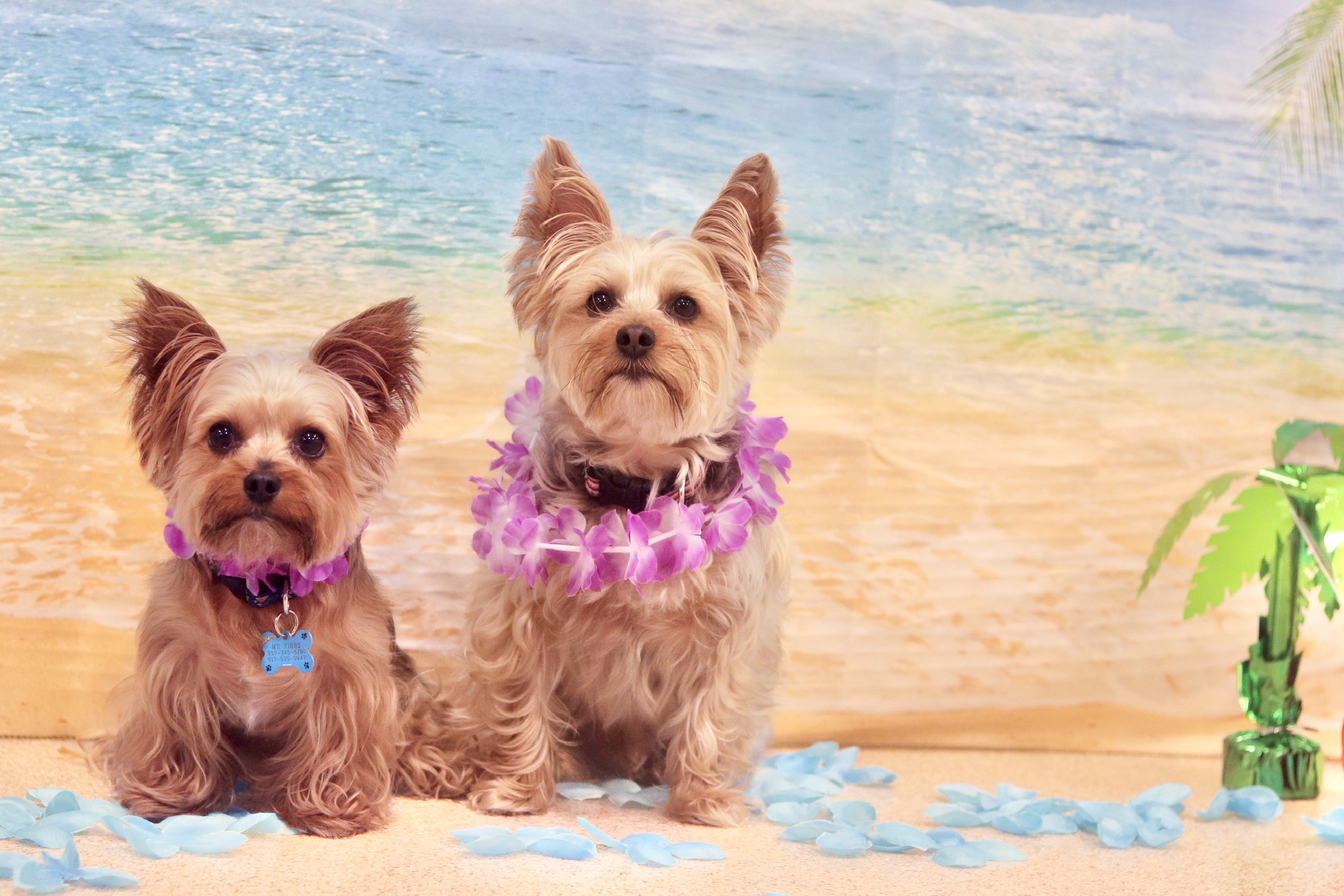This image captures a glamorous and adorable scene featuring two charming Terrier dogs, likely Yorkshire or Boston Terriers, posing against a picturesque beach backdrop complete with sand, surf, and clouds. Both dogs are adorned with vibrant Hawaiian leis around their necks, featuring petals in shades of pink with white accents. Light blue flower petals are scattered beneath their feet, enhancing the tropical aesthetic. The dogs are situated in the lower left corner of the image, with a synthetic green palm tree to their right, adding to the vacation ambiance. One Terrier is slightly larger than the other, suggesting a possible age difference or natural variance in size. The larger dog on the right and the smaller one on the left both wear black collars; the dog on the left also sports a blue bone-shaped tag. Both dogs gaze attentively at the camera, their little pointy ears, scruffy beards, and tan and white fur giving them an irresistibly cute appearance, ready for their close-up in this whimsical, beach-themed portrait.